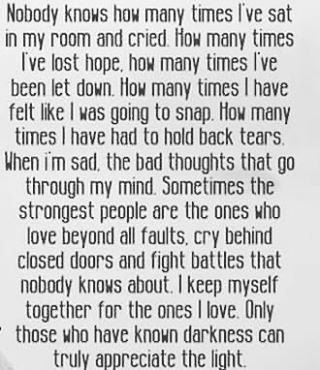The image showcases a motivational and emotional quote against a grayish-white, slightly worn background. The text is written in slim black font and spans the full length and width of the image. The message reads: "Nobody knows how many times I've sat in my room and cried. How many times I've lost hope, how many times I've been let down, how many times I've felt like I was going to snap, how many times I have had to hold back tears when I'm sad. The bad thoughts that go through my mind. Sometimes the strongest people are the ones who love beyond all faults, cry behind closed doors, and fight battles that nobody knows about. I keep myself together for the ones I love. Only those who have known darkness can truly appreciate the light." This image appears like a social media post, perhaps shared on platforms like Instagram or Facebook, meant to offer comfort and support to those who feel alone. The text is accompanied by subtle shadowing that adds depth to the somber yet inspirational message.